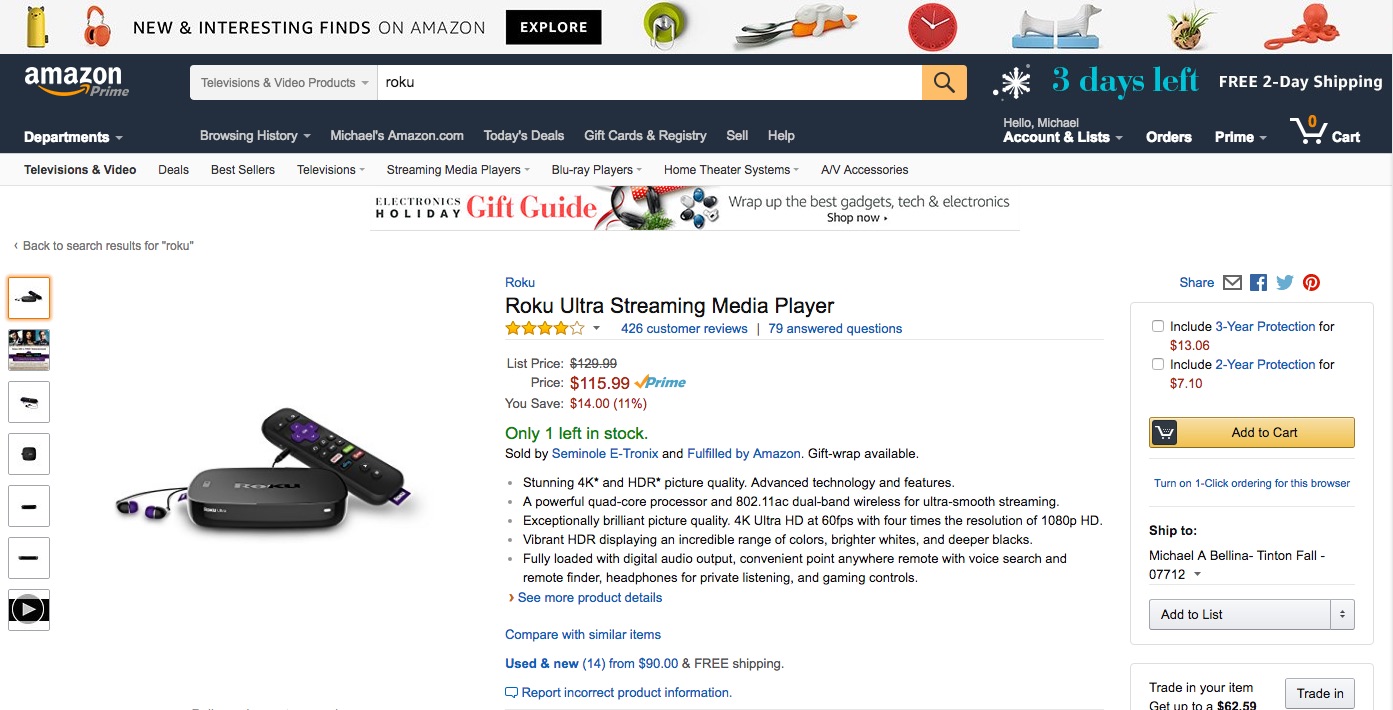A computer screen displays the Amazon website. At the top of the page, a vibrant banner showcases an array of diverse products under the tagline "New and Interesting Finds on Amazon," with an "Explore" button inviting users to discover these new items. Directly below this, the standard Amazon banner is visible, featuring the familiar "amazon.com" logo on the left and a prominent search bar. In the search bar, the user has specifically searched for "televisions and video products," particularly items related to Roku.

To the right of the search bar, an emblematic snowflake icon draws attention, accompanied by a prompt that reads "3 days left for Free Two-Day Shipping." The navigation menu at the bottom of the banner displays various links, including "Browsing History," "Michael's Amazon.com," "Today's Deals," "Gift Cards & Registries," "Sell," and "Help." Additionally, it shows a personalized greeting: "Hello, Michael," alongside options for "Account & Lists," "Orders," and a visible shopping cart indicating items inside.

The user has navigated to the televisions category to view relevant products. Prominently displayed is a Roku Ultra Streaming Media Player, noted to be on sale with a reduced price from $129 to $115.99. The urgency to purchase is underscored by a stock note: "Only 1 left in stock." Service protection plans for the product are available for either three or two years, which can also be added to the cart before proceeding to checkout.